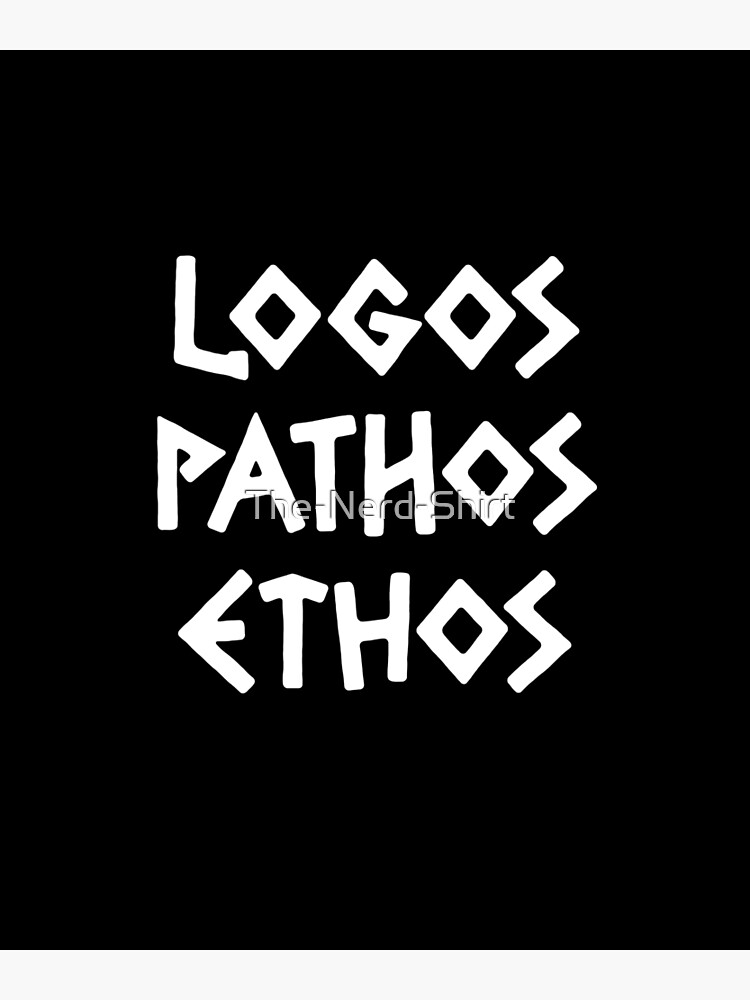The image features a black background with white text positioned diagonally in the center. The text, which appears jagged and reminiscent of Greek lettering, consists of three lines. At the top is "LOGOS," followed by "PATHOS" in the middle, and "ETHOS" at the bottom. The letters exhibit distinctive shapes: all the O's resemble diamonds, the S's look like zigzags or lightning strikes, and the P, T, and H in "PATHOS" have slanted sections. The Z in the S's are particularly jagged. Additionally, the E in "ETHOS" appears as a sideways L with a horizontal line. At the very center of the image, there is a watermark reading “The Nerd Shirt” in an off-white silver color, blending seamlessly with the unique font style and adding to the design's cohesive look.